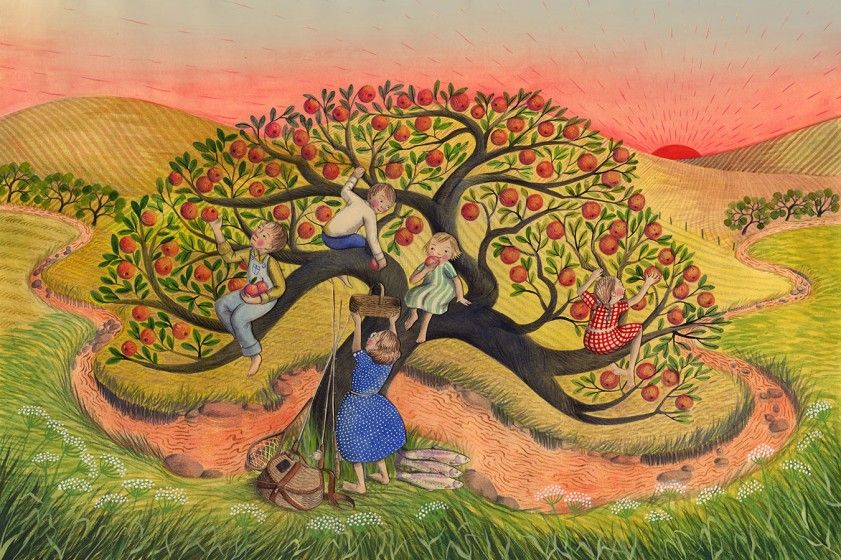This whimsical drawing, reminiscent of children's book illustrations, captures a tranquil scene set in a grassy prairie field under a sky transitioning from red at the horizon to gray at the top. At the center is a large apple tree laden with red apples. Four children, dressed in various garments—girls in dresses and boys in long pants, all barefoot—are engaged in picking the apples. Two boys are seen on the left side of the tree, while two girls are on the right, one notably in a blue dress handing a basket to a boy. Another girl, dressed in red, sits on a branch gathering apples as well.

Below them, a woman, possibly their mother, stands in a blue dress, collecting apples in a basket. Scattered around her feet are fishing gear and three rainbow trout, hinting that the group has been fishing earlier. The idyllic scene is accented by a meandering stream with ducks, visible in the foreground. On the field's rolling hills, there are a couple of paths meandering through the tall grass, leading towards distant trees and the sun, which is ambiguously either rising or setting. This enchanting and serene moment is devoid of any signatures or text, focusing purely on the timeless joy of outdoor family activities.